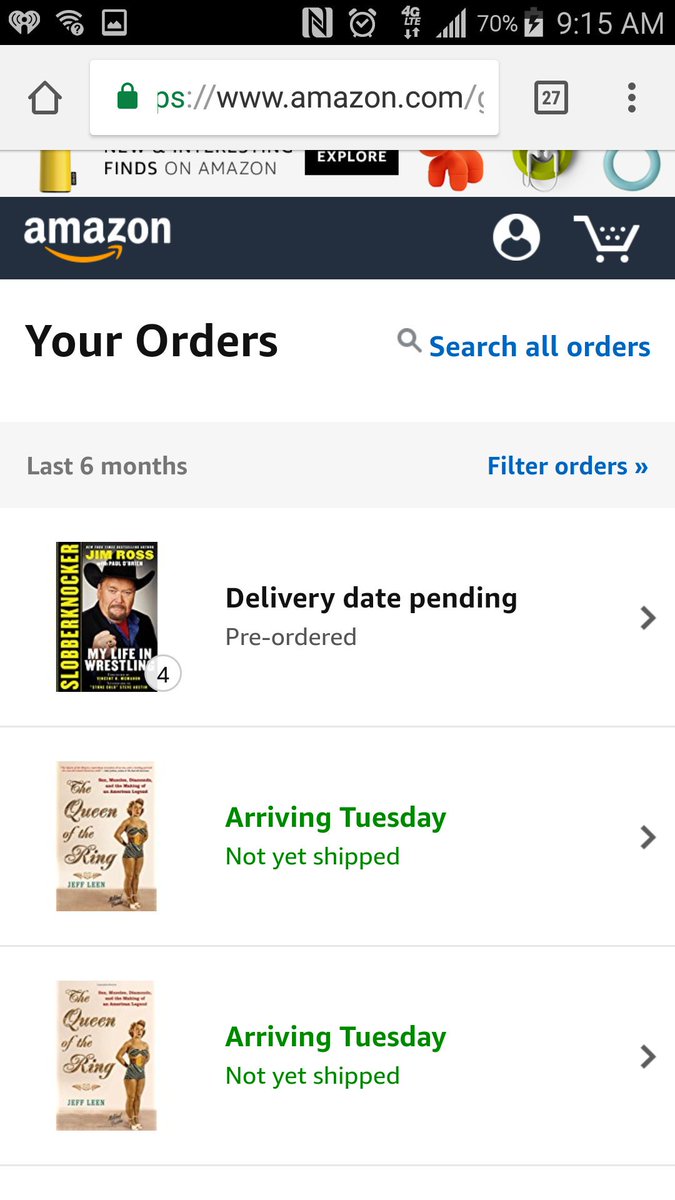The image is a screenshot of an Amazon order history page displayed on a mobile device at 9:15 a.m., with the battery level at 70%. At the top of the screen, there are several recognizable icons, including a profile logo and a shopping cart.

The page prominently features a search bar with a magnifying glass icon, allowing users to search through their past orders. Below the search bar, there are hyperlinks for "Search all orders" and "Filter orders," both highlighted in blue. The filter is set to display orders from the last six months.

The order history displays several statuses including "Delivery Date Pending," "Pre-order," and "Arriving Tuesday." The image shows there are four items expected to arrive on Tuesday, with at least one item marked as "Not yet shipped," indicated in green text. The background of the page is completely white, providing a clean contrast to the text and icons.